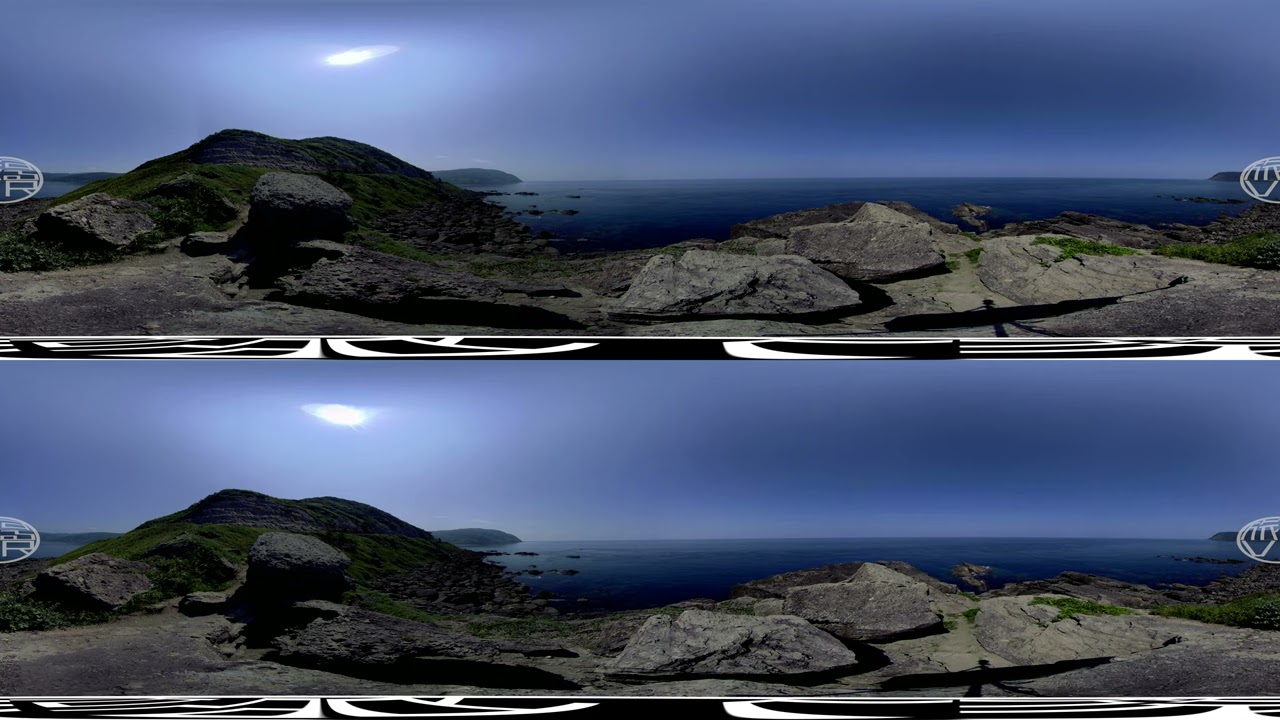This panoramic image, featuring a duplicated landscape stacked vertically, offers a mesmerizing view of a serene natural scene. The predominant feature is a deep, calm blue ocean stretching towards the horizon, dotted with small islands. In the foreground, large moss-covered rocks dominate the scene, transitioning into a rocky shoreline with patches of green vegetation. A hill on the left side gradually descends into the rocky coastal area continuing to the right. The entire scenery is bathed in bright sunlight under a clear, cloudless blue sky. Additionally, subtle details like logos, likely indicative of digital artwork, are present on the far right and left edges of the image, completing a composition that seamlessly blends natural beauty and artistic elements.